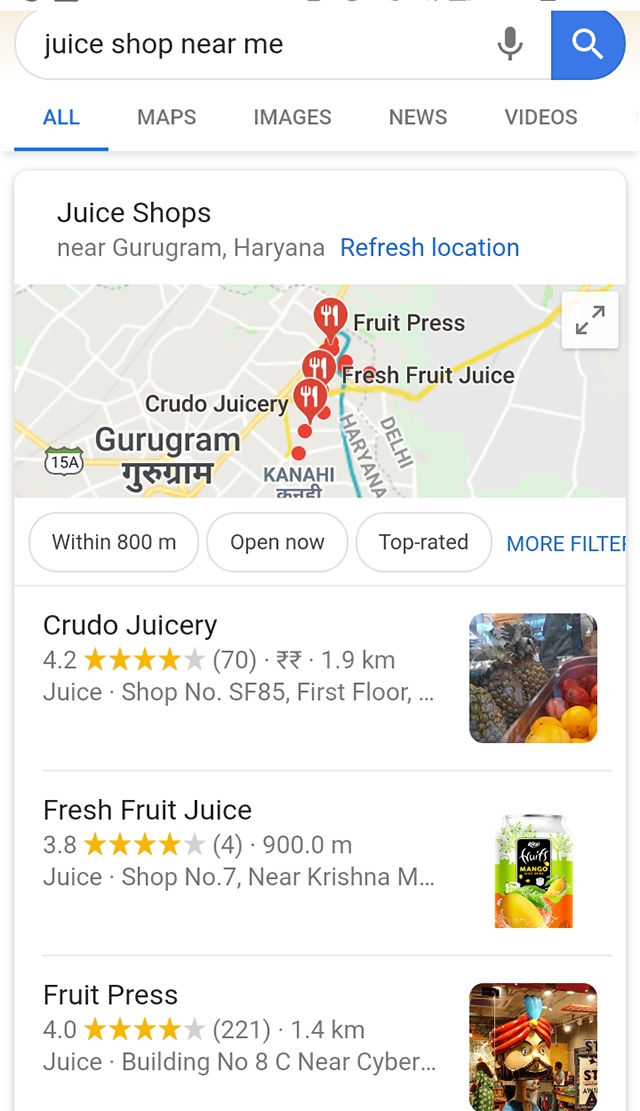This screenshot appears to be from a mobile device, displaying search results for "juice shop near me". At the top of the screen, there's a search bar with the input text "juice shop near me," accompanied by a microphone icon to its right and a search button further to the right.

Below the search bar, there are category tabs labeled "All," "Maps," "Images," "News," and "Video." The "All" tab is highlighted in blue, indicating the current selection. The primary section of the screen displays a map titled "Juice shops near Gurugram, Haryana," with the option to "Refresh location" in blue text on the right.

On the map, various points are marked, pinpointing locations such as "Fruit Press" and "Fresh Fruit Juice." Beneath the map, there are filter options labeled "Within 800 meters," "Open now," and "Top rated," with a "More filters" button in blue text on the right side to access additional filtering options.

Following the map and filter options, three juice shops are listed with their respective ratings, review counts, and distances from the user's location:

1. **Crudo Juicery** – Rated 4.2 stars with 70 reviews, located 1.9 kilometers away.
2. **Fresh Fruit Juice** – Rated 3.8 stars, located 900 meters away.
3. **Fruit Press** – Rated 4.0 stars, located 1.4 kilometers away.

This detailed search result layout helps users quickly identify and choose from popular juice shops in Gurugram, Haryana.